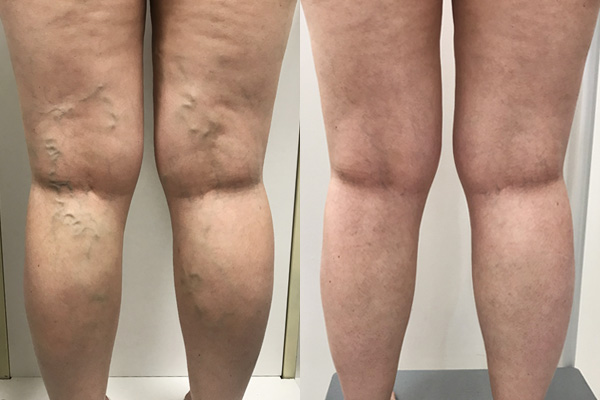The image displays a side-by-side comparison of the back side of a pair of light-skinned legs, likely Caucasian, taken from just above the knees down to almost the ankles. In the left photograph, the legs are shown with visible blue varicose veins, especially behind the knees, along with some spots and bumps. The right photograph depicts the same legs after an evident medical procedure, now free of varicose veins, with clear and smooth skin. The images are set against a white wall, with the person standing on a gray floor mat or surface in front of it. The comparison clearly highlights the efficacy of the varicose vein removal or treatment.